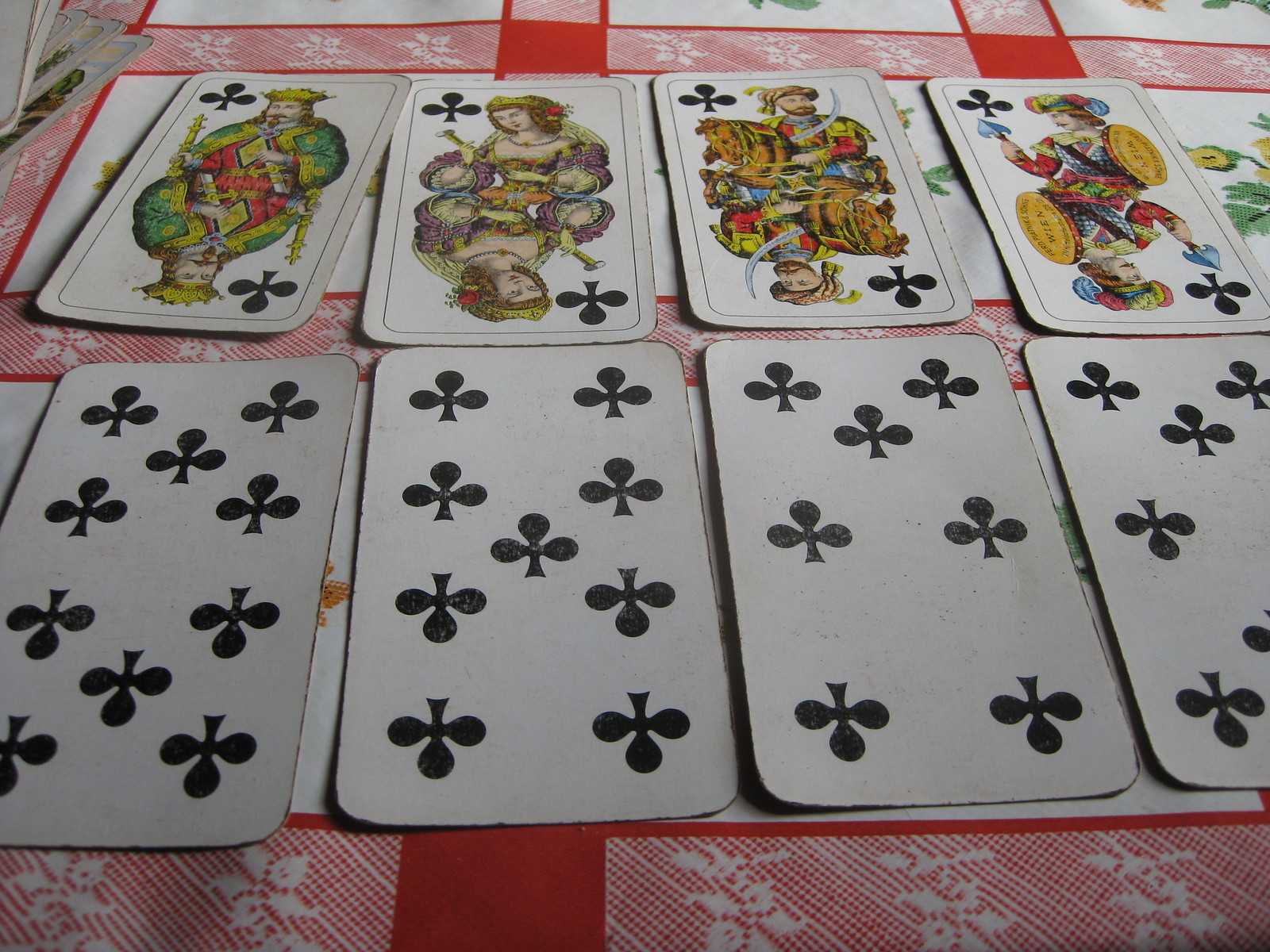The image depicts an arrangement of playing cards laid out on a surface with a red and white tablecloth. There are two rows of cards, each containing four cards. In the top row, all the cards belong to the suit of clubs, identifiable by their black, clover-like symbol. The first card is a King of Clubs, featuring the illustration of a king with a mirrored reflection. The second card is a Queen of Clubs with a similar mirrored design. The third and fourth cards in the row also appear to represent members of aristocracy, though their specific identities are not clear.

The bottom row consists of four cards that also display face cards or other significant symbols. The overall impression is that of a formal and classic card game setup, with vibrant touches provided by the red and white tablecloth underneath. The detailed imagery and placement of the cards convey an elegant, timeless atmosphere, despite the viewer’s unfamiliarity with card games.